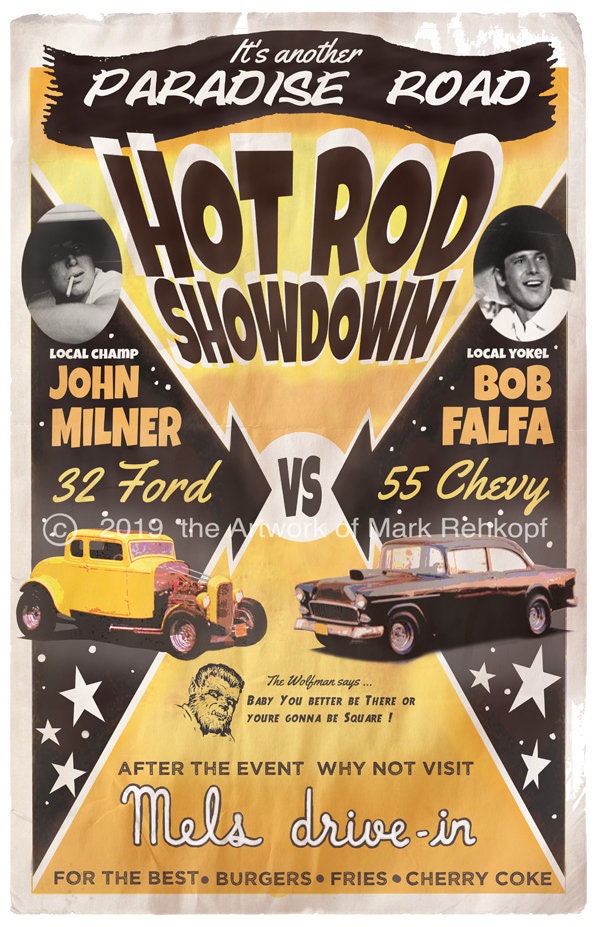This promotional poster, bathed in vintage-inspired yellow and dark brown hues, advertises the "Another Paradise Road Hot Rod Showdown." Featuring prominently in the design are two iconic hot rods: a yellow '32 Ford Roadster with a massive engine and fat tires, labeled as driven by the local champ, John Milner, who is depicted in a nostalgic black-and-white photo, smoking a cigarette. To the right, grinning slightly away from the camera, is the local yokel, Bob Falfa, associated with a formidable black '55 Chevy Bel Air, his name emblazoned in striking yellow letters. A quote from the Wolfman urges, "baby, you better be there or you're gonna be square." The poster, adorned with a copyright watermark by Mark Reckhoff from 2019, invites spectators to the high-stakes showdown and suggests a post-event visit to Mel's Drive-In for the best burgers, fries, and cherry coke.